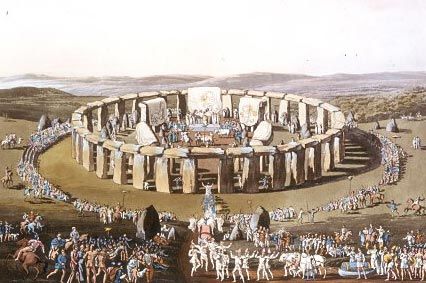This detailed illustration, likely a historic depiction or a creative imagining of Stonehenge, features an iconic stone circle at its center. The structures, consisting of upright stones with horizontal lintels, dominate the scene, surrounded by bustling crowds. Within the stone circle, people gather too small to discern individual activities, except for some visible white banners or sheets draped over internal structures. Encircling this central congregation, another large group of people forms an outer ring. Among them are individuals on horseback and clusters dressed in various attire, including white garments, while others appear unclothed. The scene conveys a sense of ancient ritual, highlighted by a lively front group, possibly dancing. The background stretches out into low-lying mountains or hilltops, with hints of a body of water and scattered trees on the right, set against an otherwise flat, grassy plain. The entire illustration, painted in daylight, offers a vivid and expansive view of this enigmatic gathering at Stonehenge.